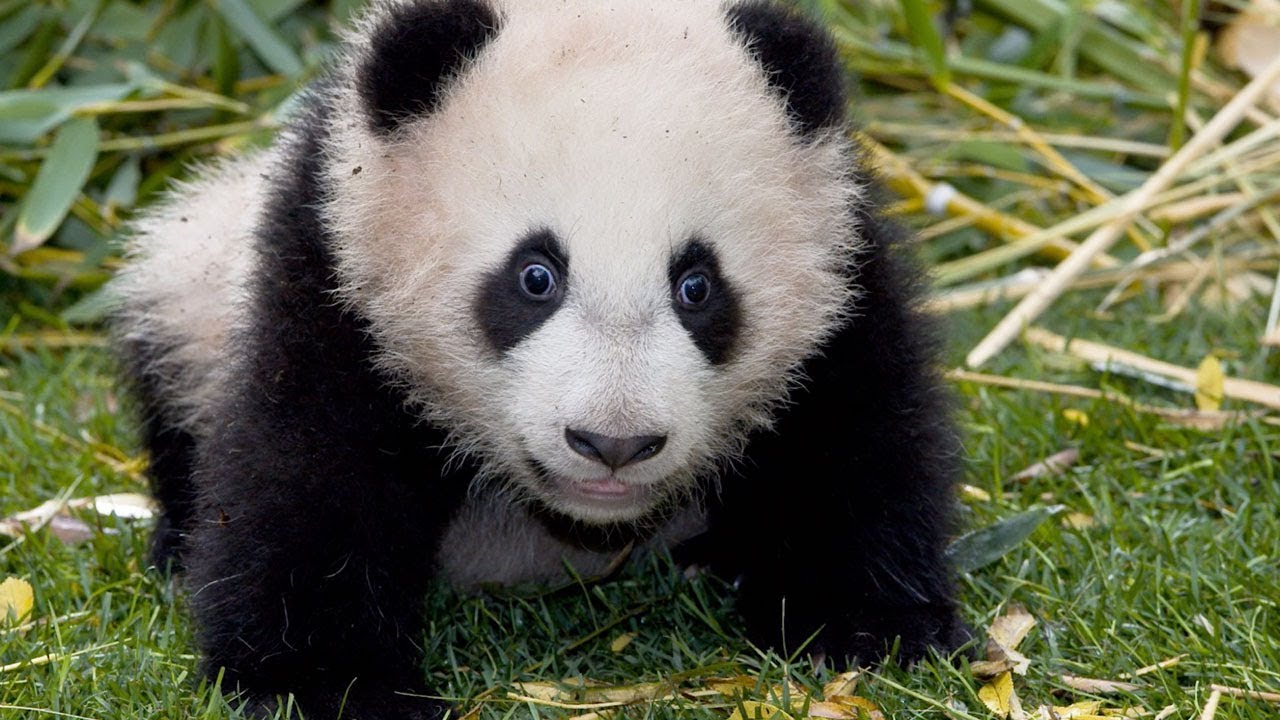This detailed photograph captures an adorably startled baby panda standing on all fours amidst a grassy area dotted with yellow leaves. The small panda faces the camera directly, its wide eyes giving it a surprised expression, intensified by its slightly open mouth and barely visible tongue. Its white face and body contrast sharply with its black ears, eyes, arms, legs, and nose. The fur appears a little dirty, with clumps of dirt sticking to its hair, enhancing its endearing charm. Surrounding the panda is an assortment of bamboo—both dead and vibrant green—adding a rich, natural backdrop to the scene. The vivid greens of the grass and bamboo plants accentuate the panda's striking black-and-white fur, making it the adorable focal point of the image.